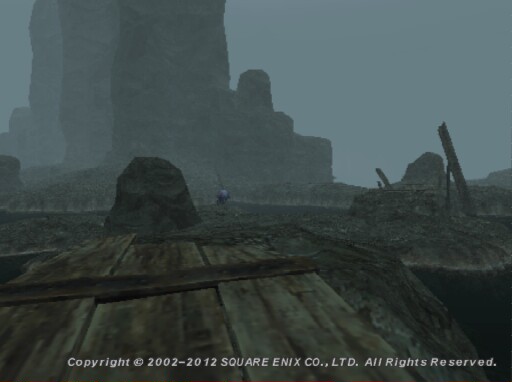In this atmospheric game scene from Square Enix, towering dark gray rock formations, etched with intricate lines, stretch into the distance. The stony ground below mirrors the rugged texture of the rocks above. The overcast sky casts a somber, grayish hue over the landscape. In the foreground, a prominent mound of rock can be seen on the right, partially encircled by a moat-like body of water that adds depth to the scene. A weathered wooden board, reinforced with a strip of metal, lies across the water, with sections extending to the left, middle, and right. This immersive visual is underscored by the copyright notice at the bottom, reading "© 2002-2004 square-enix.co., ltd. All Rights Reserved."